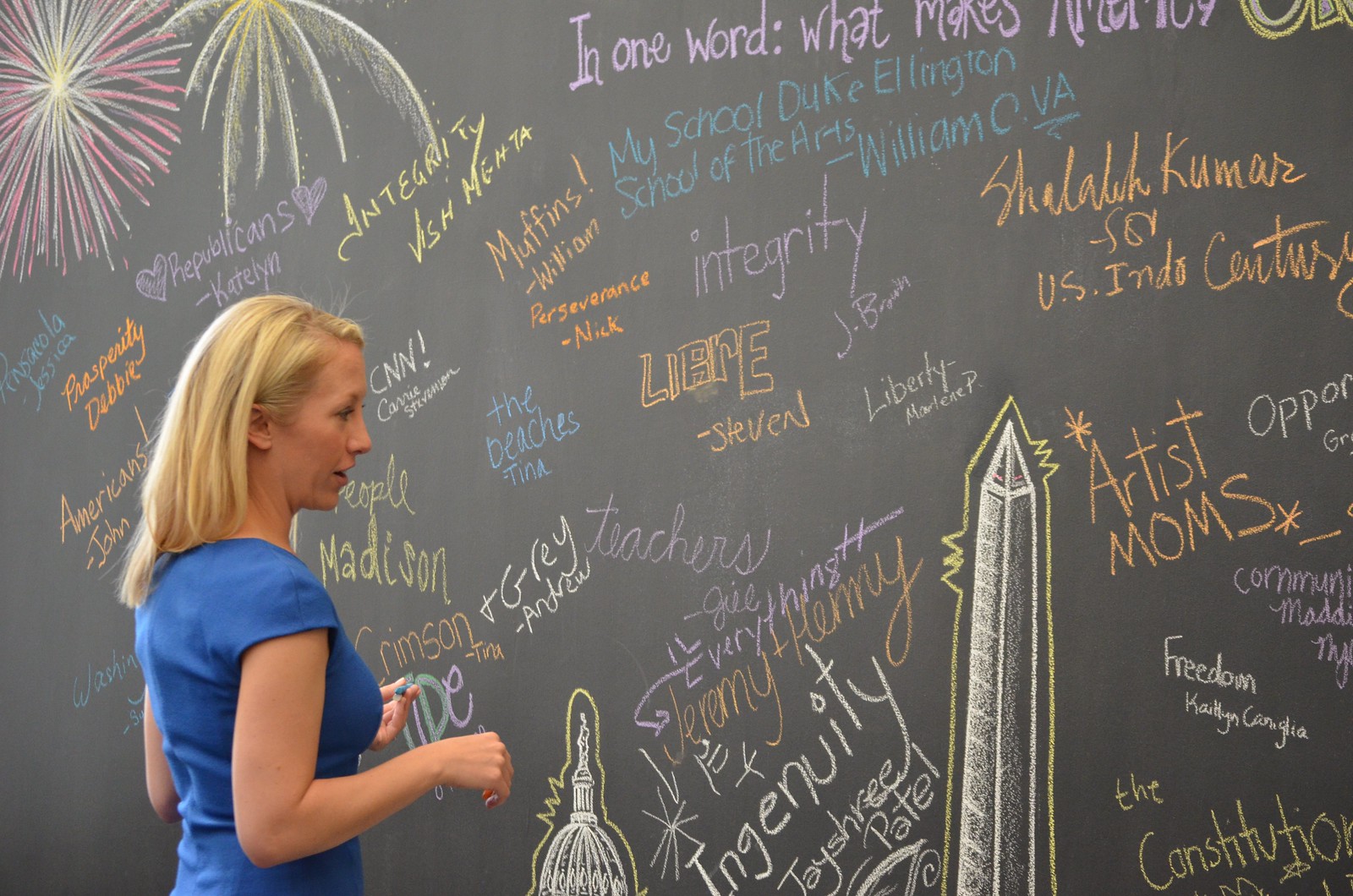The image depicts a classroom scene with a large, colorfully inscribed black chalkboard as the backdrop. At the forefront on the left side, there is a young, blonde-haired teacher, identifiable as a white woman dressed in a blue short-sleeve shirt, standing and facing the chalkboard while holding a piece of chalk. The chalkboard is covered in an eclectic mix of words and drawings in various colors, including pink, blue, orange, and white. Some of the legible words and phrases include "Integrity," "My School, Duke Ellington School of the Arts," "Liberty," "Freedom," "Prosperity," "The Constitution," and names like "Caitlin," "Larry," "Steven," and "Jessica." Additionally, detailed drawings adorn the board, such as fireworks in pink, white, and yellow at the upper left corner, and sketches of the Washington Monument and the Capitol Dome in the lower part, highlighted with yellow outlines. The chalkboard's collage of text and imagery creates a vibrant and dynamic visual representation of thoughts and ideas, all framed by the instructor's active presence in the classroom.